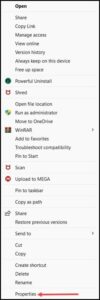The blurry image depicts a right-click context menu typically seen in desktop operating systems. The menu has a white background and lists various actions that can be performed on a selected file or item. At the top of the menu, the option "Open" is visible. Following this are several other commands including "Copy link," "Manage access," and "View version history." 

Further down, the menu includes options such as "Always keep on this device," "Free up space," and an entry with a green icon labeled "Powerful something." Additionally, the term "Shared" appears, possibly indicating shared file settings. 

Other options present are "Open file location," "Run as administrator" (accompanied by a small administrator icon), "Move to one something," and "WinRAR." The menu also lists "Add to favorites," "Troubleshoot," and an entry with a shield icon, likely related to security scans. 

Subsequently, the menu includes "Upload to MEGA," "Pin to taskbar," "Copy as something," followed by standard actions like "Send to," "Cut," "Copy," "Create shortcut," "Delete," "Rename," and "Properties," which is marked by a red bar icon next to it.